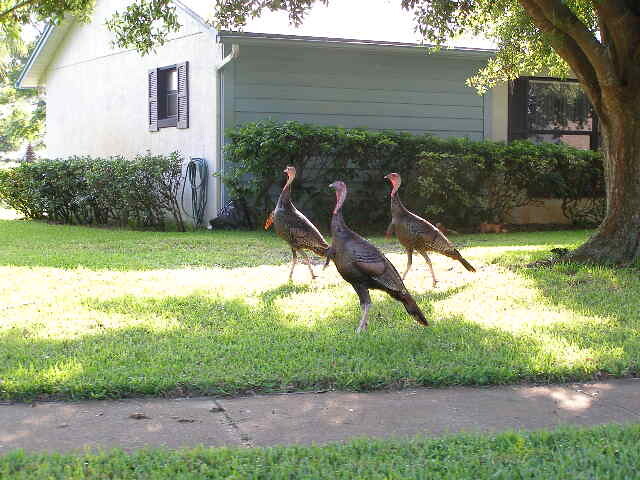In this outdoor photograph, three wild turkeys take center stage as they stroll confidently through a sunlit yard. The yard, typical with its lush green summer grass, is divided by an older sidewalk that stretches from the bottom left to the bottom right of the image. Above the sidewalk, the turkeys can be seen walking on the grass, each with a majestic presence. Their heads, reminiscent of turkeys with yellow beaks and red necks, contrast against their dark brown speckled bodies and off-white legs. Their poised strut and elegant stature almost give them the appearance of turkeys adorned in tuxedos. 

In the background, a single-story house with a light gray façade stands partially visible, adorned with gray shutters and surrounded by green shrubbery. A coiled hose hangs from one corner of the house, adding a touch of everyday detail. To the right of the house, a tree trunk and branches provide shade to parts of the yard, enhancing the composition. The clear, sunny day casts a gentle light, bringing out the textures and colors of this quiet, suburban scene.